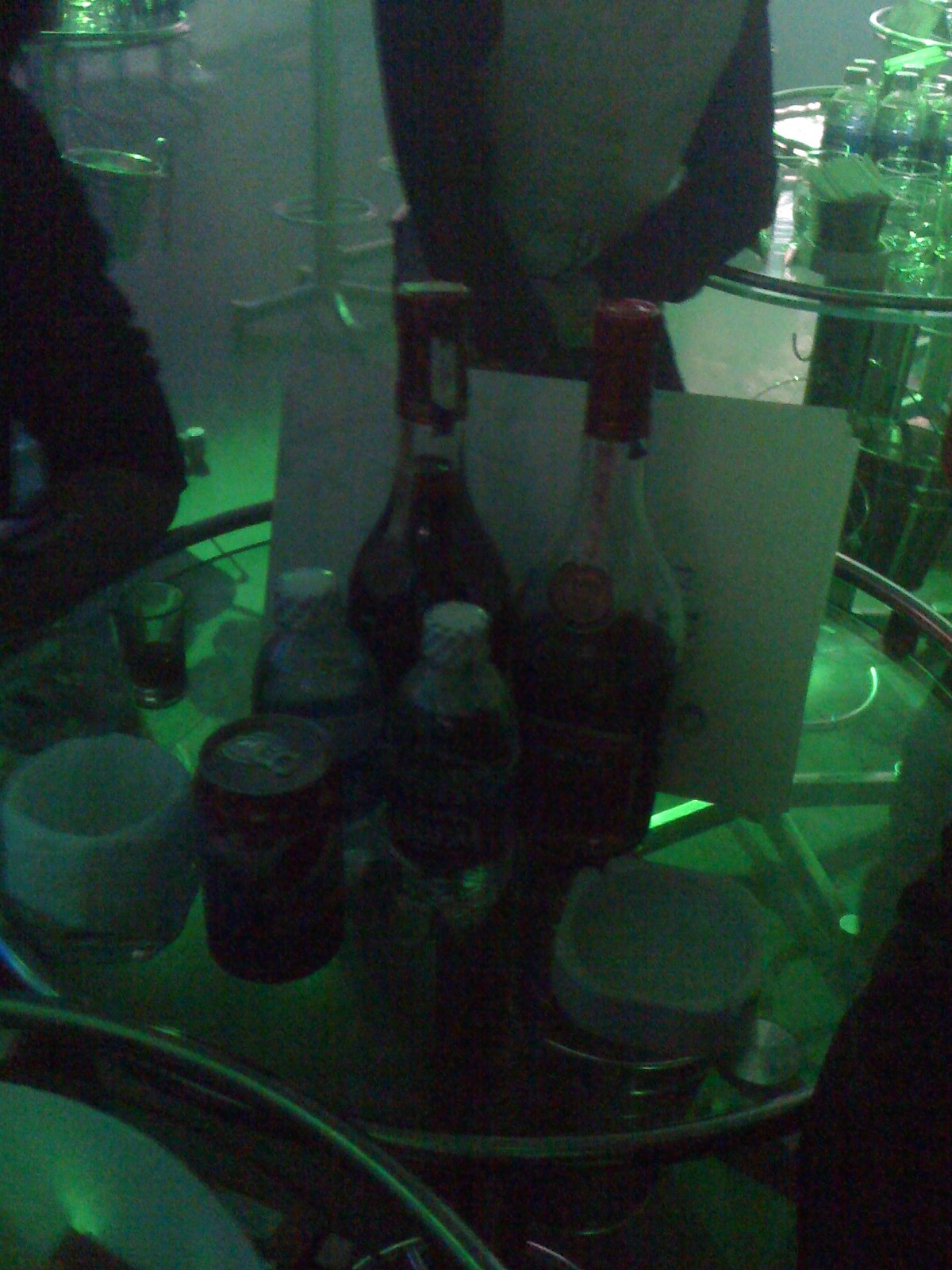In this dimly lit and grainy image, likely captured in a nightclub or bar, a circular glass table supported by a metal frame holds an assortment of items. The table is illuminated by green neon lighting, which casts a hazy glow over the scene. Among the items on the table are two large bottles resembling whiskey or brandy, two smaller bottles that could be mixers or water, and a can drink situated towards the front. There is also a shot glass and possibly a white candle. Additional details include an ashtray and a piece of paper in the background. The image lacks clarity due to the absence of a flash, making it difficult to discern specific details. However, the presence of dark, shadowy figures and another glass table in the background suggest it was taken in a busy nightlife setting.